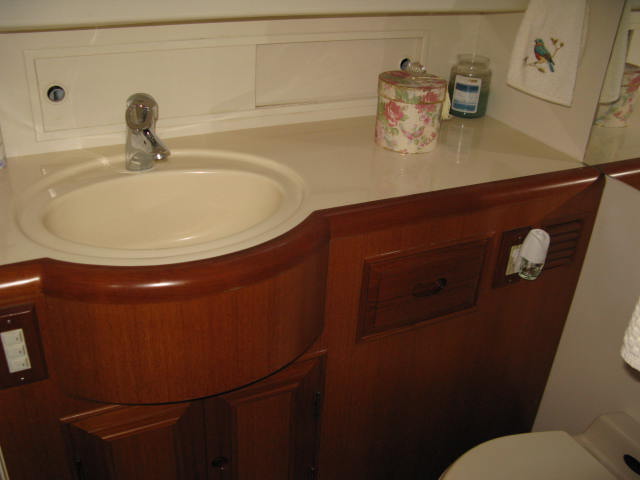The close-up image showcases an exquisitely designed bathroom hand wash basin and its elegant countertop. The sink, crafted from lustrous white porcelain, possesses a flawless circular shape that exudes sophistication. The countertop, which boasts a remarkable sheen, reflects the various items placed upon it, adding to the room’s opulent feel. It features a unique design with a curved extension at the center, seamlessly cradling the circular sink. The countertop and accompanying cabinetry are constructed from polished wood with a rich brown hue, accented by a subtle red tint, enhancing its luxurious appearance. Additionally, the picture captures a glimpse of a mirror’s edge on the wall, as well as the edge of a toilet seat, hinting at the cohesive design elements throughout the bathroom.